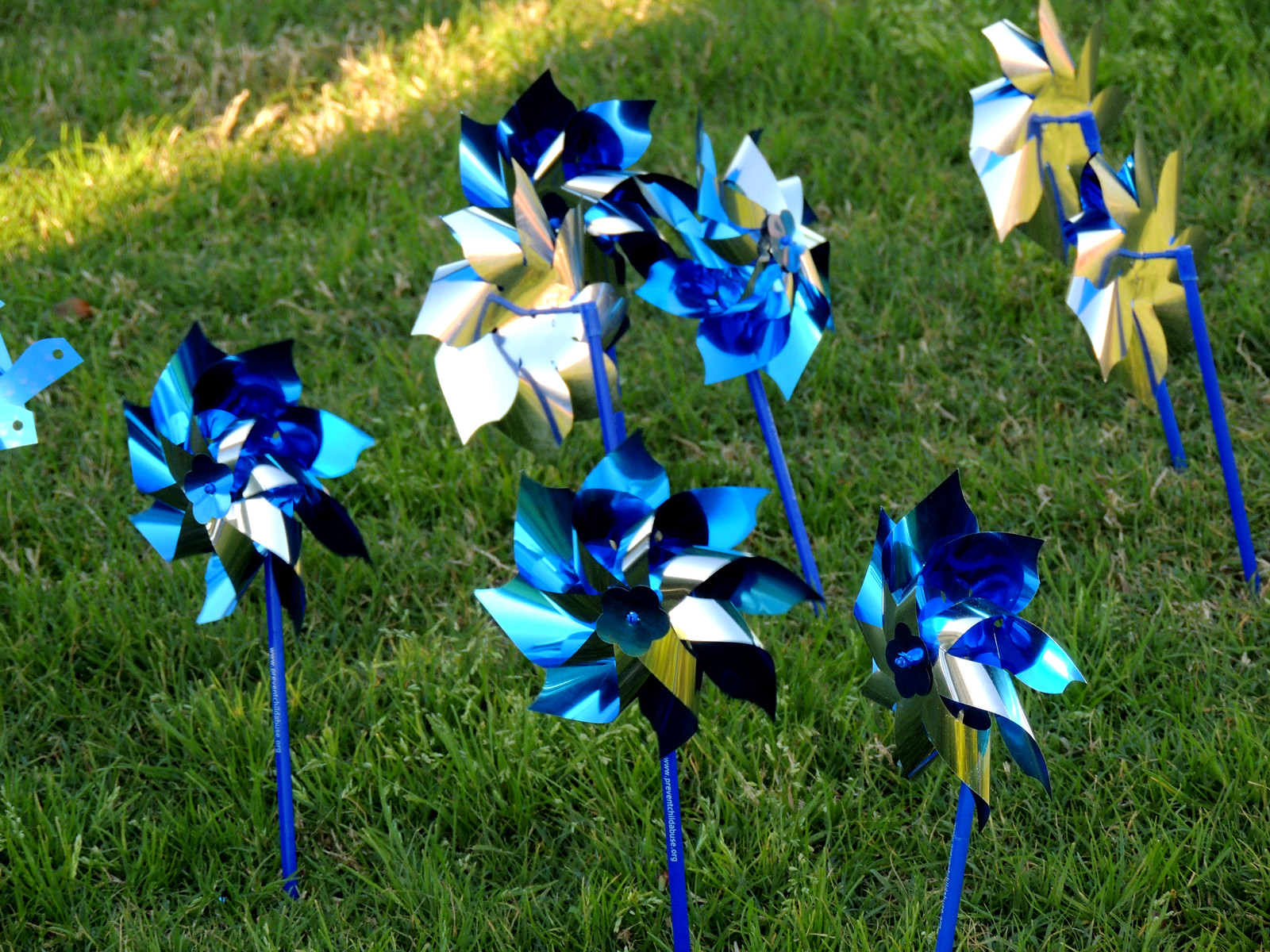This photograph captures approximately ten pinwheel spinners, installed in a lush green lawn. The pinwheels stand out with their bright metallic blue fronts and silvery backs, appearing to be made of thin, flexible material like plastic or aluminum foil. Each pinwheel is mounted on a slender blue stake, firmly planted into the grassy ground. The configuration of the pinwheels shows some facing different directions, creating a dynamic feel as if they're ready to spin with the slightest breeze. The scene is set under gentle daylight, as evidenced by a narrow streak of sunlight cutting diagonally across the top of the image, while the rest of the lawn remains in a comfortable shade. The well-organized placement of the pinwheels is notable, with three in the middle, two at the bottom foreground, one at the bottom left, and two more at the top right, adding to the picturesque quality of the landscape.